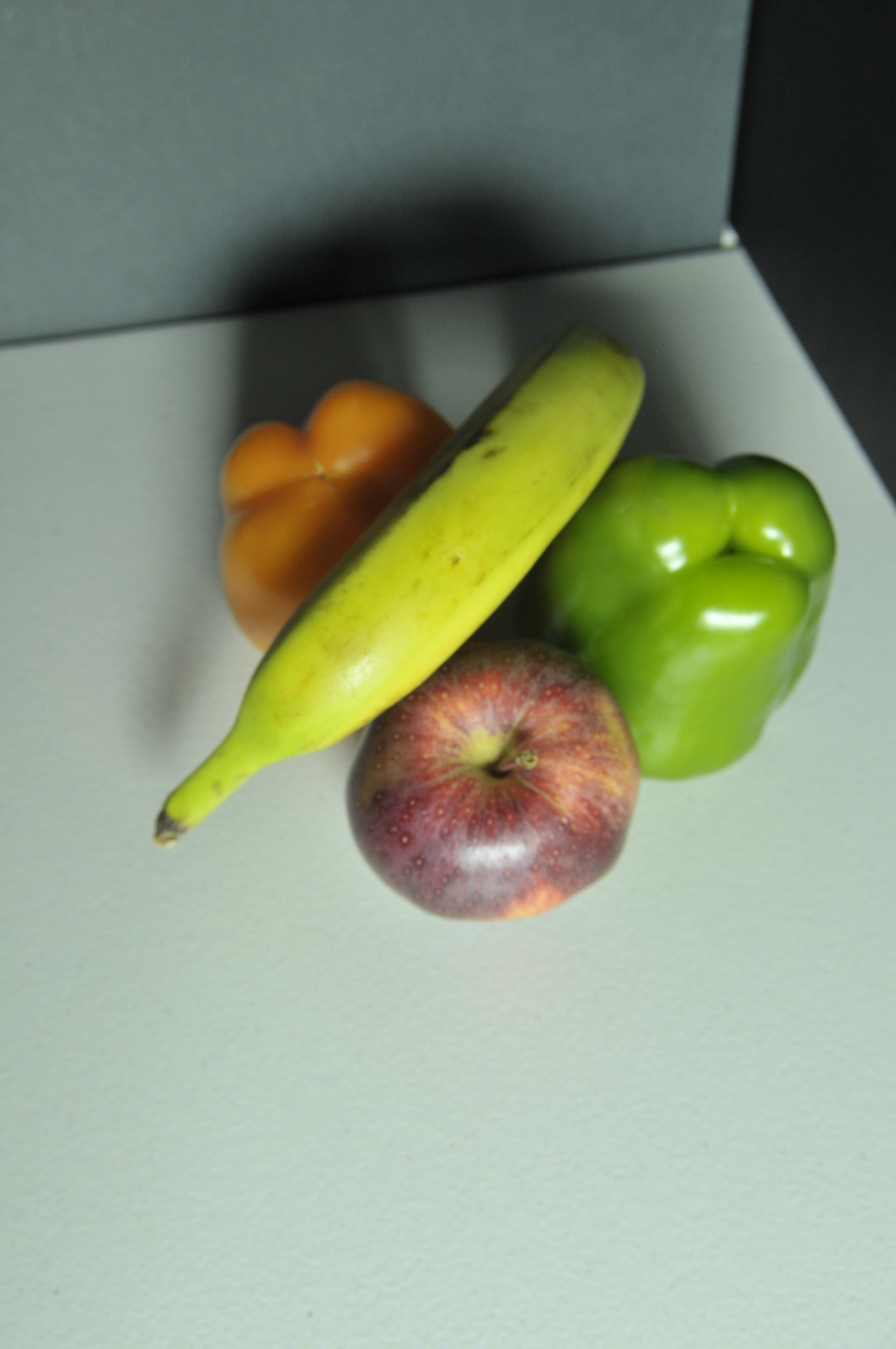This overhead photograph captures a vibrant assortment of fruits and vegetables arranged in the corner of a light gray counter. The backdrop includes a darker gray wall behind the produce and a black wall to the right. Central to the arrangement is a slightly mottled but ripe red apple with its stem still attached. Flanking the apple are two glossy bell peppers, one green and one orange, positioned bottom-up. Completing the composition, a ripe banana with minimal green near the stem and some bruising on its left side arches gracefully over the apple and peppers.